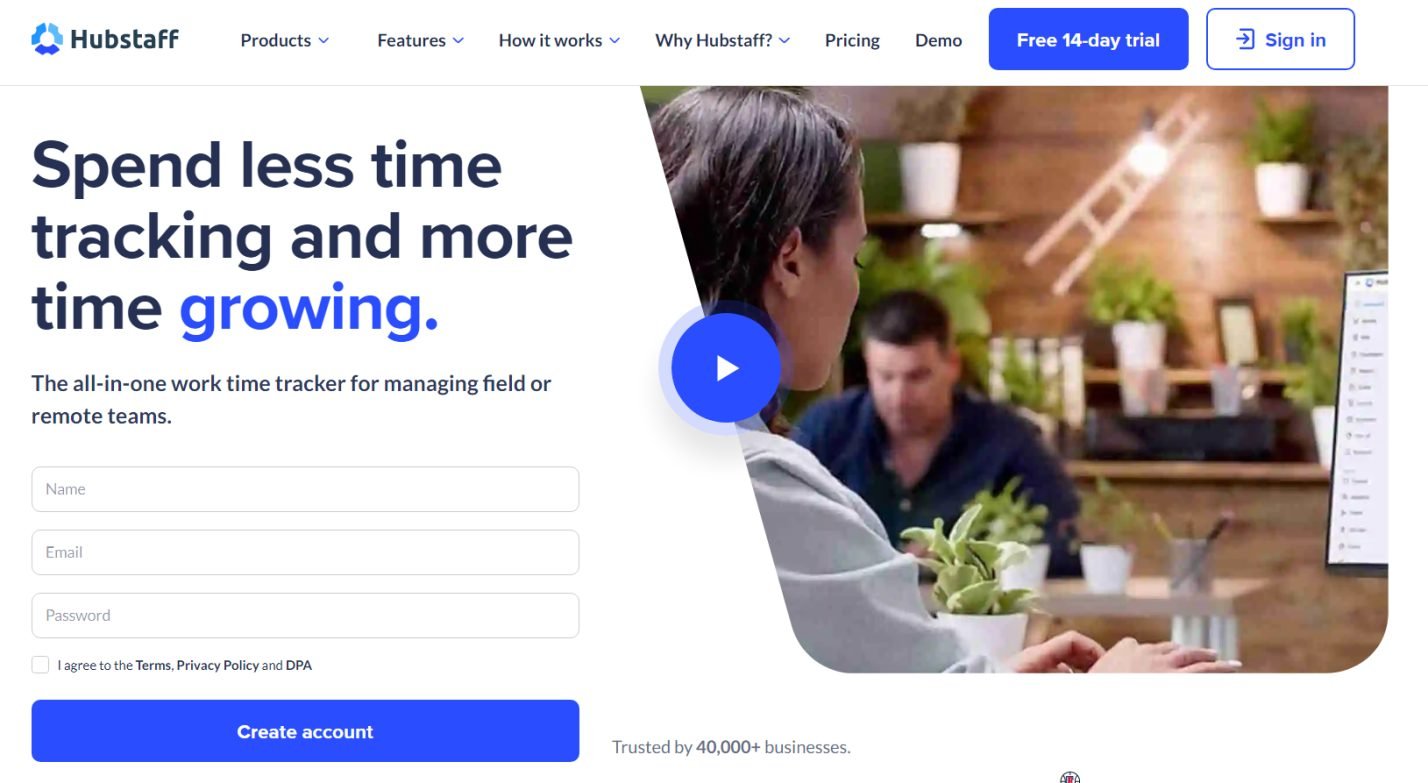Screenshot of the Hubstaff website's homepage. In the upper left-hand corner, the Hubstaff text is accompanied by their logo, which features a combination of navy blue and light blue hues. To the right of the logo, a navigation menu spans the top of the screen, including options labeled "Products," "Features," "How It Works," "Why Hubstaff," "Pricing," and "Demo." Adjacent to these menu items are two buttons: a blue button with white text that says "Free 14-Day Trial," and a white button with blue text that says "Sign In."

Below this navigation bar, the tagline reads, "Spend less time tracking and more time growing." In a smaller font beneath it, there is a description that states, "The all-in-one work time tracker for managing field or remote teams." Directly below this tagline, input fields are presented for users to enter their name, email, and password. There is also a checkbox for agreeing to the terms and conditions. Below these fields, a blue button with white text instructs users to "Create Account."

To the right of the input fields is a bold statement highlighting the platform's credibility: "Trusted by 40,000+ businesses." Adjacent to this, an image features two individuals: a partially visible woman working on her computer in the foreground, and a man in the background, seated at his desk and also engaged in work. The scene portrays a professional and collaborative work environment, reinforcing the utility of Hubstaff for managing both field and remote teams.